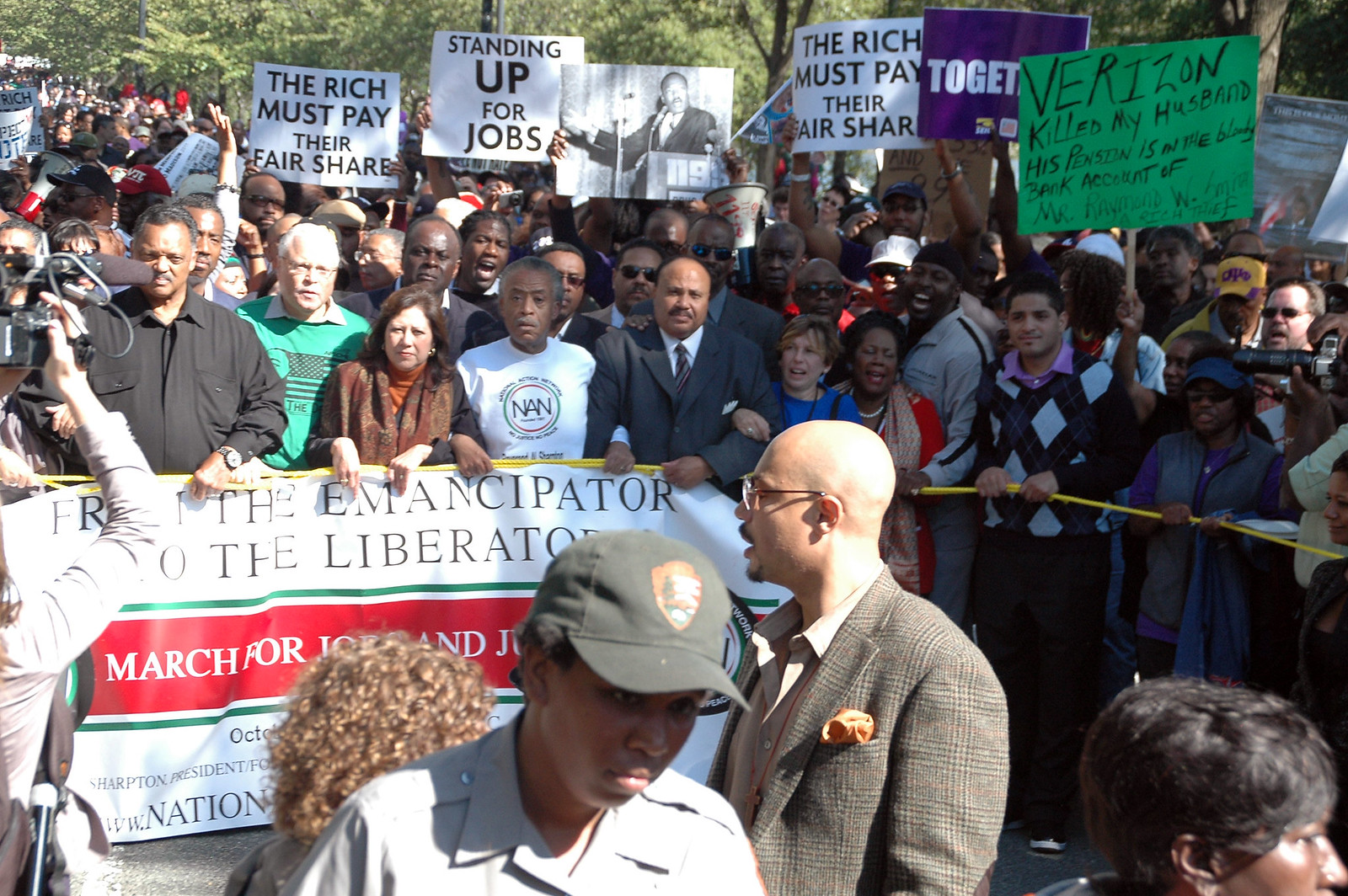The image depicts a large protest rally filled with a diverse crowd of men and women of various age groups. The protesters are gathered behind a yellow rope barrier, holding an assortment of placards with messages such as "The Rich Must Pay Their Fair Share" and "Standing Up for Jobs." Several signs are prominently displayed in the background, including a green one with the partially visible message, "Verizon Killed My Husband. His Pension is in the Bloody Bank Account of Mr. Raymond."

At the forefront of the scene stands a white banner with red and green elements, bearing the words "Free the Emancipator" and an incomplete phrase, "of the Liberation." Additional text on this banner remains partially obscured. 

Among the crowd, several individuals stand out: a bald man wearing glasses and a suit jacket; a person in a uniform and baseball cap with their head bowed; and a short lady with curly blonde hair. A cameraman, equipped with a mic, captures the event from the left corner of the image. 

The atmosphere is charged, with loudspeaker mics and flags contributing to the vibrancy of the protest, as demonstrators passionately advocate for economic justice and employment rights.